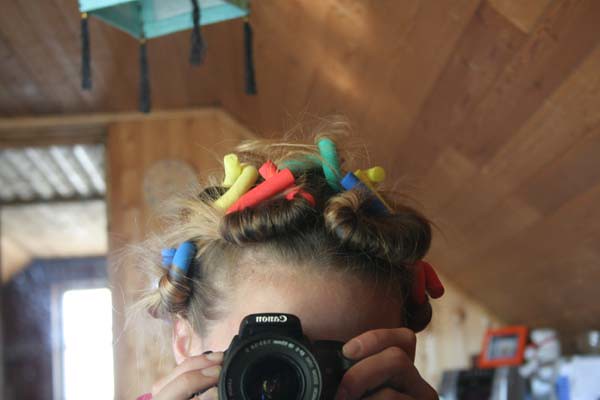The image captures a young female taking a photograph of herself in a mirror, as evidenced by the reversed Canon logo on her camera. She is positioned in what appears to be a wooden cabin with an octagon-shaped ceiling, featuring light brown wooden panels. The girl's hair is styled with multicolored sponge curlers—blue, yellow, red, and green—adding a playful touch to her appearance. Above her hangs a box with black tassels at its four corners, adding an element of decor. The sunlight streams through a window in the far left corner, illuminating parts of the space. While her facial features are obscured by the camera, her hands and the upper portion of the Canon camera are in clear view. In the background, there's a teal-colored lamp and some blurred objects, including a photo frame, contributing to the cozy, lived-in atmosphere.